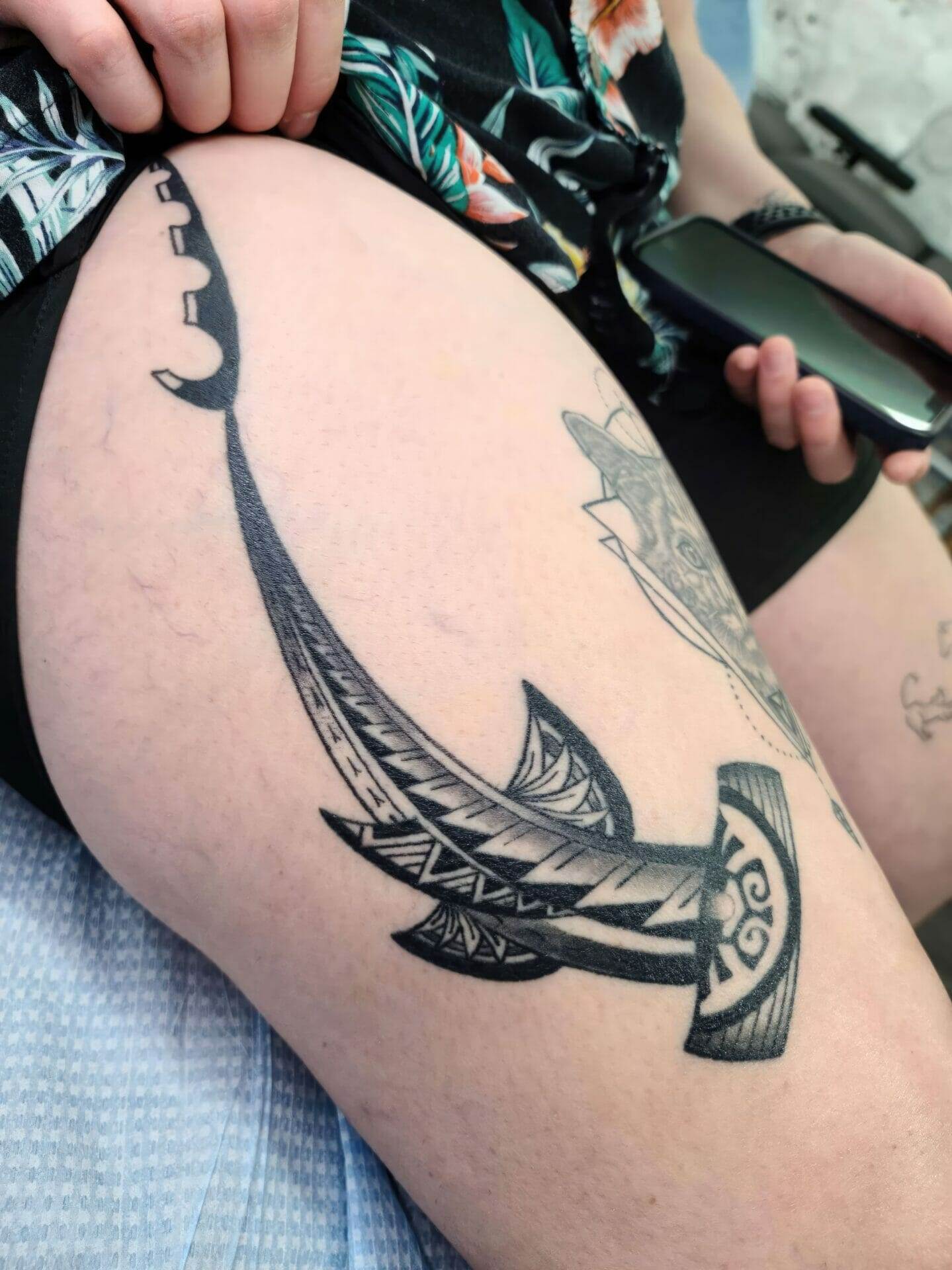This image depicts a person lifting their black shorts to reveal a detailed tattoo on their right thigh, prominently featuring a black and white hammerhead shark. There is another partially hidden tattoo on the right leg, with only a portion visible, suggesting additional intricate designs. The left thigh also bears a tattoo that is not clearly discernible. The individual appears to be holding a black cell phone in their right hand, and perhaps a watch or bracelet wraps around their left wrist. They are dressed in a black shirt accented with a vibrant mix of green, yellow, orange, and white hues. The setting seems to be a tattoo studio, indicated by the blue and white paper towel-like mat beneath their legs. The background is nondescript, featuring gray and white elements. The overall atmosphere is focused on the person's legs and tattoos, set against a backdrop of various colors including blue, white, black, green, yellow, and orange.